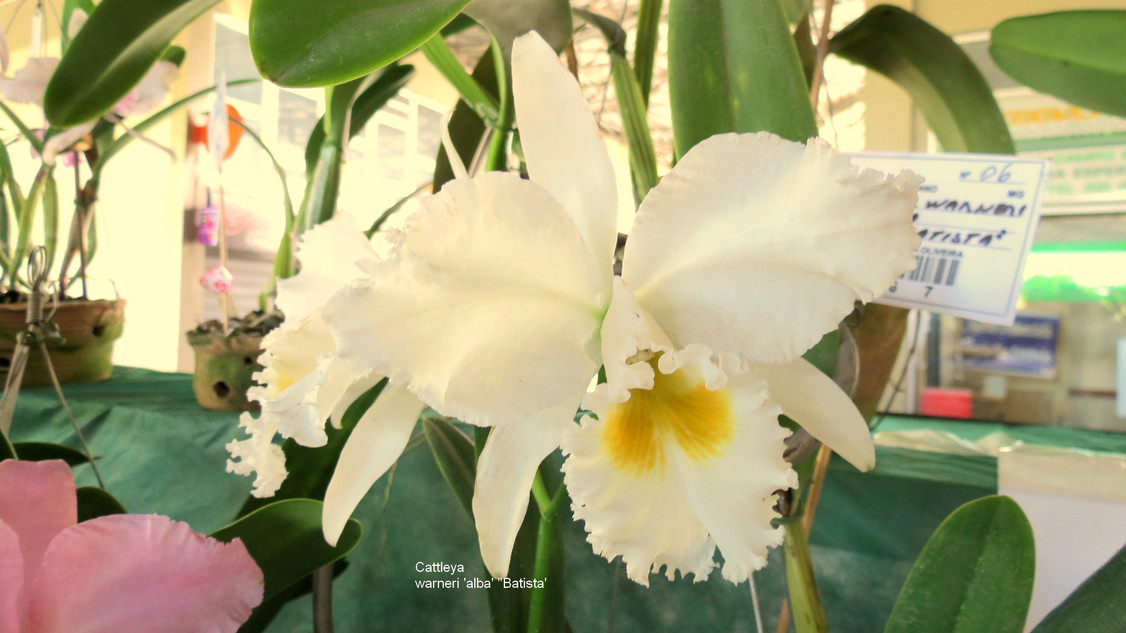This photograph features a delicate white flower with a vibrant golden-colored interior, identified as Catalaya Warnari Alba Batista, likely its scientific name. The petals are fragile, contrasting with the thick, vibrant Kelly green leaves beneath them. The flower appears to be in a well-lit area, evidenced by the glowing light yellow background. In the bottom left corner, pink petals from another flower suggest the presence of another species nearby. Additionally, a few potted plants can be seen in the background, although it's uncertain if they belong to the same genus or species. This detailed composition highlights the intricate beauty and vivid colors of the flora.